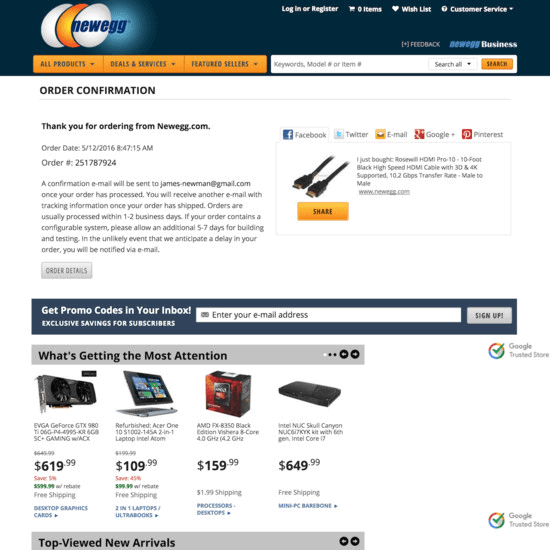This detailed caption illustrates the features and elements of a Newegg website page, specifically an order confirmation screen:

---

The Newegg website features a user-friendly interface tailored for purchasing electronic items. The top navigation bar includes options for logging in, registering an account, viewing the shopping cart (currently empty), accessing a wishlist, and a customer service drop-down menu. The Newegg logo comprises three tilted ovals (white, orange, and white) with the word "Newegg" inscribed in the final oval.

An orange bar below the logo offers categories such as "All Products," "Deals," "Services," and "Featured Sellers," while a prominent search box allows users to find items using keywords, model numbers, or item numbers.

Displayed on the screen is an order confirmation, thanking the user for their purchase made on May 12, 2016, at 8:47:15 AM. The confirmation email has been sent to jamesnewman@gmail.com. The notice details that the user will receive tracking information via email once the order is processed within one to two business days, with additional time required for configurable systems.

To the right, a customer review highlights the purchase of a Rosewill HDMI Pro 10-foot black high-speed cable, which can be shared on social platforms like Facebook, Twitter, Google+, and Pinterest. Users can also opt to receive promotional codes via email.

The bottom section features popular items, including refurbished laptops and modems, and top-viewed products, all showcased on an all-white background with colorful images. The site is identified as a Google-trusted source, and the topmost section has a dark blue background highlighting the "NUIC" and "All Products" categories.